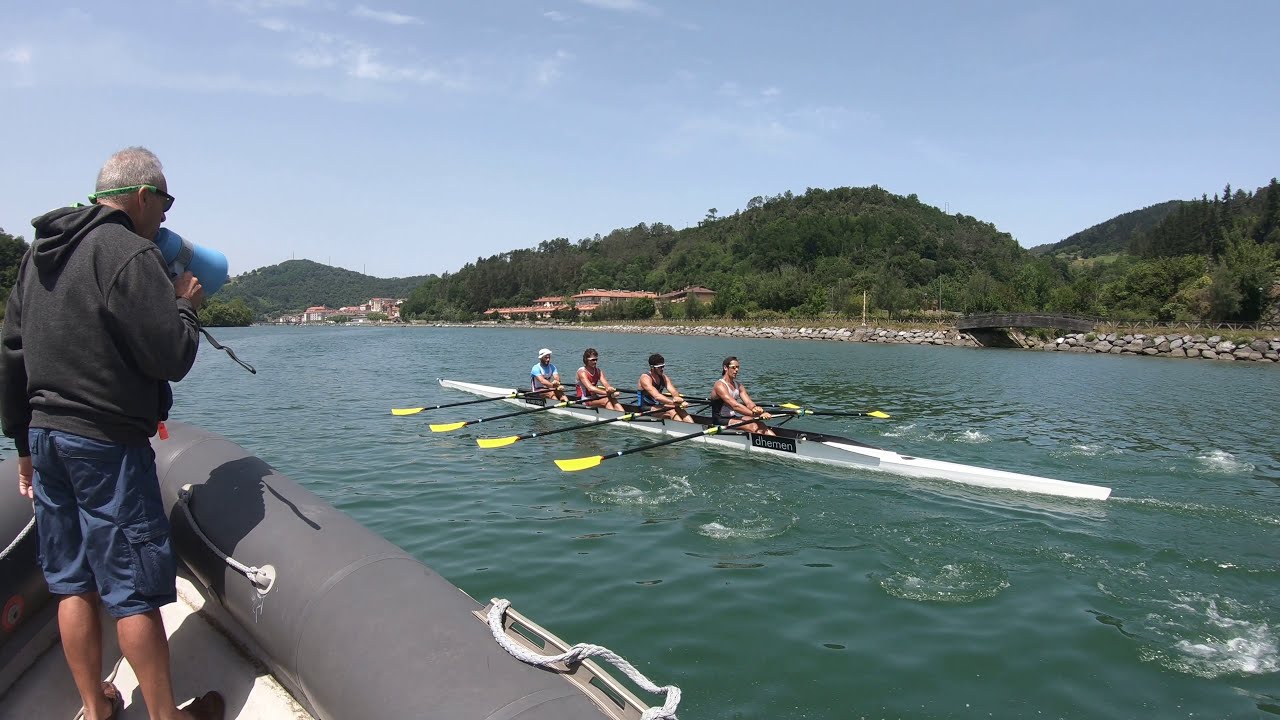In this vibrant and dynamic scene, a rowboat team of four is fiercely paddling down a stretch of greenish-blue water under a sunny, blue sky dotted with a few wispy clouds. The team consists of three men and one woman, all in tank tops, with the man at the back wearing a blue shirt and a white hat. They are in a sleek, thin white boat, using black-handled oars with bright yellow paddles. Amidst the white and foamy water stirred by their oars, a gray-edged inflatable boat powers alongside. In this larger boat, a coach dressed in navy blue shorts, a black hoodie, and sunglasses uses a blue megaphone to urge the rowers to push harder, shouting, "Row, row, row!" On the right-hand side, the shoreline is lined with rocks forming a barrier, and in the distance atop the rolling, green vegetated hills, a red-roofed house peeks out. The scene captures the intense and competitive spirit of the rowers as they strive towards their goal, driven by their coach's passionate encouragement.